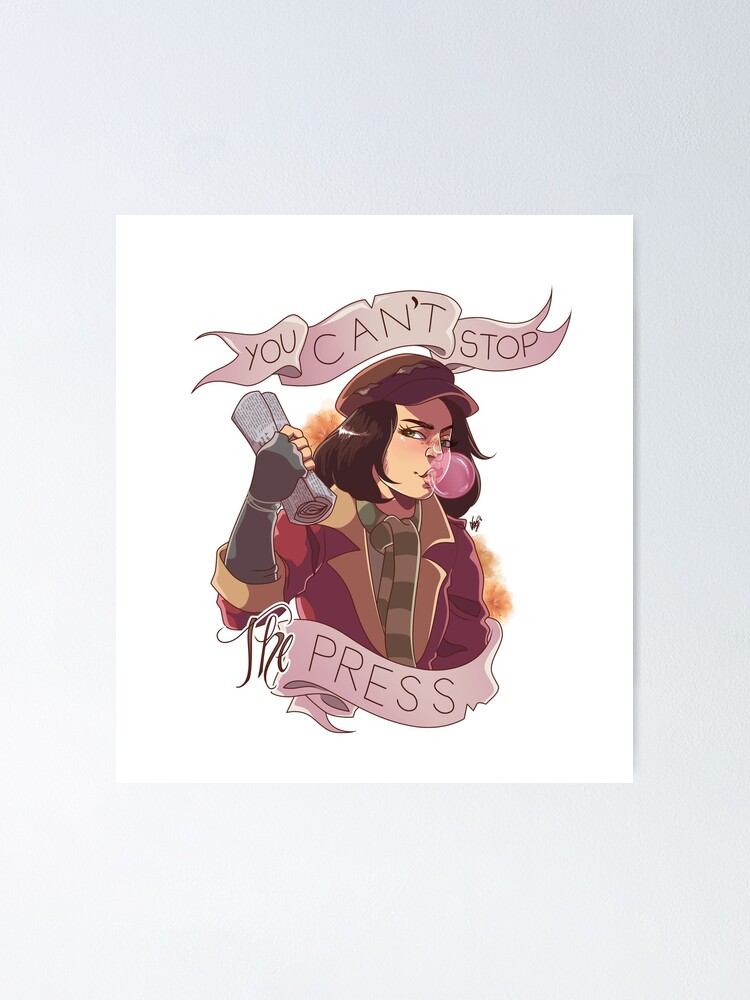The image showcases a detailed digital illustration on white background featuring a young woman against a blue-lit backdrop. She has short brown to black hair and dons a newspaper boy cap. She is depicted blowing a pink bubblegum while holding a rolled-up paper in her right hand. She is dressed in a pink coat, light and dark green striped scarf, and fingerless gloves. Above her head, a pink ribbon banner reads, "You Can't Stop," and below her body, another pink ribbon states, "The Press." This colorful scene, predominantly in shades of pink, green, and brown, conveys a dynamic, cartoon-like aesthetic with a succinct and impactful message.